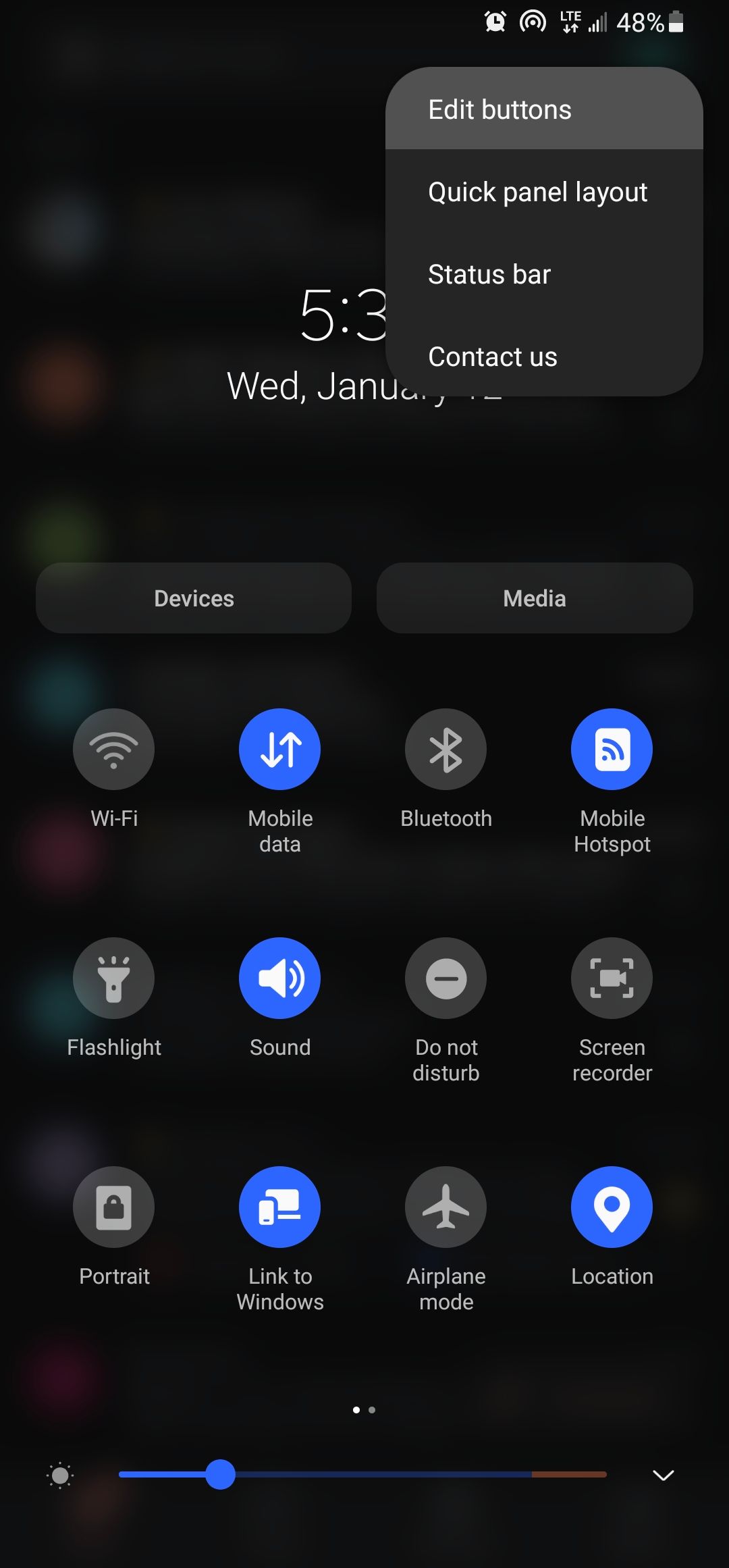The image is a detailed screenshot of a cell phone with a black background. 

In the top right-hand corner, small icons are displayed: an alarm clock, a Wi-Fi symbol, "LTE" with up and down arrows, four signal bars, and a battery icon showing 48% next to the percentage. 

Centered below is a square interface. At the top of the square, a light gray horizontal rectangle reads "Edit Buttons" in white text. Below, a black background features white text with labels: "Quick Panel Layout," "Status Bar," and "Contact Us" at the bottom.

Near the center of the image, partly cut-off text shows the number 53, "WED, January," followed by truncated content. 

Further down, two buttons are visible: "Devices" on the left and "Media" on the right. Below these, four buttons are arranged from left to right: a Wi-Fi button, a highlighted mobile data button with up and down arrows, an unhighlighted Bluetooth button, and a highlighted mobile hotspot button.

On the mid-left side of the screen is an unhighlighted flashlight icon. Right next to it is a highlighted sound button. Further right, there's an inactive "Do not disturb" button and an inactive screen recorder button.

At the bottom left, there’s a "Portrait" button not highlighted. Moving right, there's a highlighted "Link to Windows" button, an inactive "Airplane Mode" button, and a highlighted "Location" button. Finally, at the very bottom is a brightness adjustment bar, filled about a quarter of the way across.